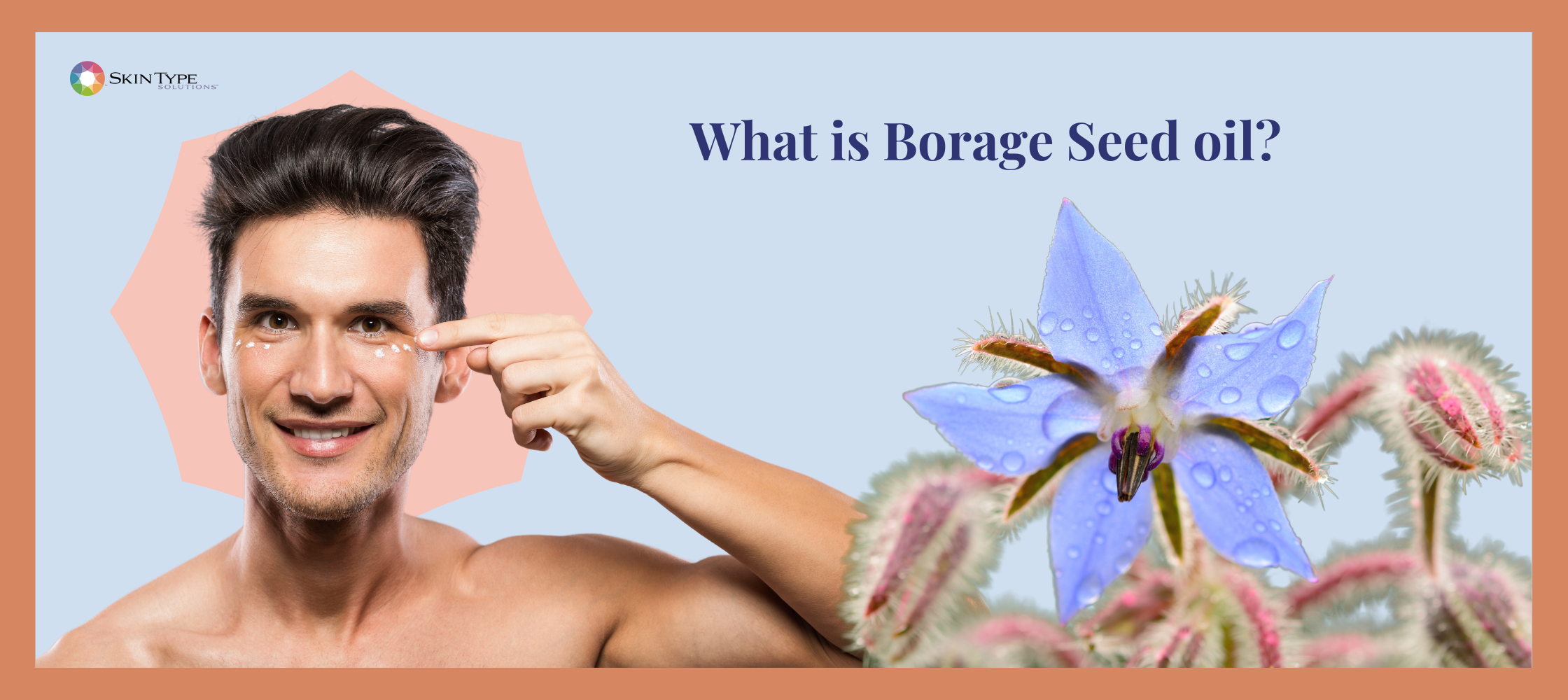The poster is a detailed advertisement featuring the question "What is Borage Seed Oil?" prominently displayed in dark blue lettering against a light blue, almost underwater-themed background. The border of the poster is a rust color, adding a contrasting frame to the soft hues within. On the left-hand side of the poster, there is an image of a well-muscled, shirtless man with brown hair slicked back, and a slight scrubby beard, smiling with shiny skin. He has three small white dots under each eye, presumably borage seed oil, and is caught in the action of raising his left hand as if about to rub the oil on his skin. Below him, the text "skin type" is written. The right-hand side of the poster features a close-up photograph of a unique and spiky pink plant, resembling a star flower, with violet-blue petals adorned with droplets of water. Several blurred, fuzzy pink and white flowers are seen in the foreground, adding depth to the image. The elements come together to create an intriguing and visually appealing advertisement for borage seed oil.